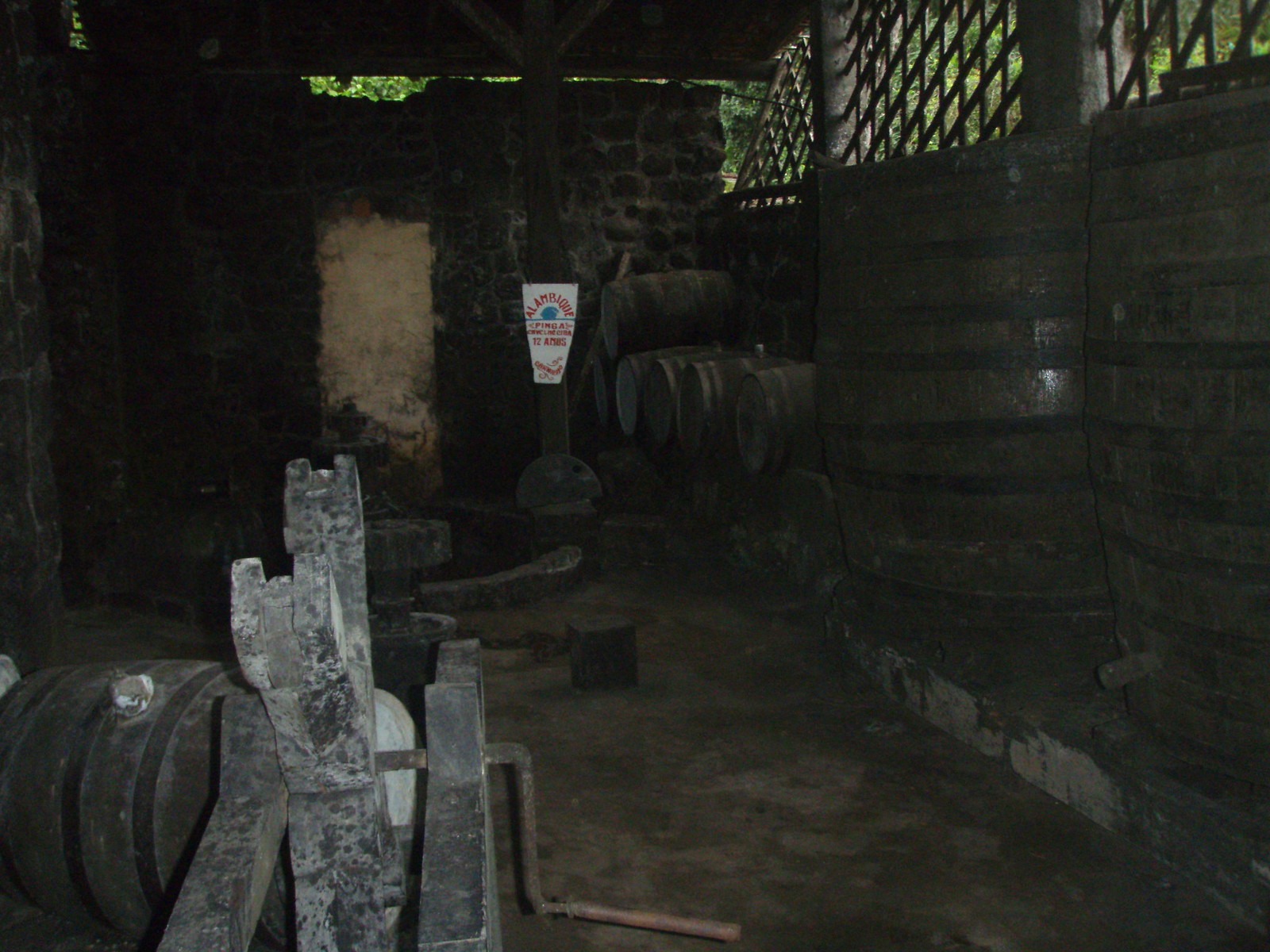This is a photograph of a dark, antiquated cellar, likely used as a wine or distillery storage area, located in the basement of a building. The scene is dominated by numerous large wooden barrels, some upright with metal rings and others lying on their sides. These barrels are scattered around, with several stacked against stone walls that form the back and sides of the room. 

The walls feature lattice openings at the top, allowing glimpses of the green trees and bright daylight outside, adding a stark contrast to the otherwise dim and dusty interior. The dirt floor is uneven, contributing to the overall disused and rustic feel of the space. 

Prominently in the foreground, there's an old, possibly antique, crank-mounted machine with tools nearby, suggesting equipment used for sealing or manipulating the barrels. A white sign can be seen off in the distance, though its text is unreadable. The setting conveys an air of age and abandonment, with various objects strewn about, evoking a sense of historical use and purpose.